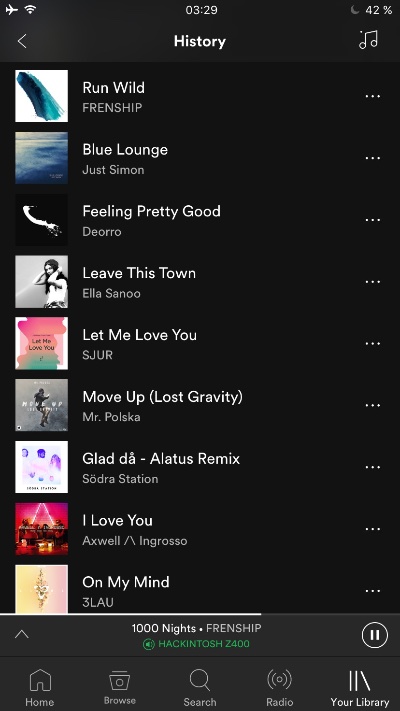This image is a detailed screenshot of someone's music history on a streaming platform, likely Spotify or Apple Music. At the very top of the screen, there's a black status bar featuring a white airplane icon, signifying airplane mode is activated. Next to it, there are three full bars of Wi-Fi signal strength, and the time displayed is 03:29. There's also a small gray half-moon icon indicating Do Not Disturb mode and a battery percentage of 42%.

Below this status bar, a white header contains a back button labeled "History" and a music icon. The main section consists of a list of nine songs, each accompanied by what appear to be the respective album covers on the left and a three-dot menu icon on the right. The listed songs are:

1. **Run Wild** by Friendship
2. **Blue Lounge** by Just Simon
3. **Feeling Pretty Good** by D'Oro
4. **Leave This Town** by Ella Sanu
5. **Let Me Love You** by SJUR
6. **Move Up** by Lost Gravity
7. **Mr. Polska** by Glad Da (Alatis Remix)
8. **Soldra Station** by I Love You (Axwell Ingrosso Remix)
9. **On My Mind** by Three Lau

Following these songs, there is an additional song listed: **One Thousand Nights** by Friendship.

Below this, there is a green label reading "Hackintosh Z400." 

At the very bottom of the screen, there is a navigation bar featuring five icons labeled: Home, Browse, Search, Radio, and Your Library.